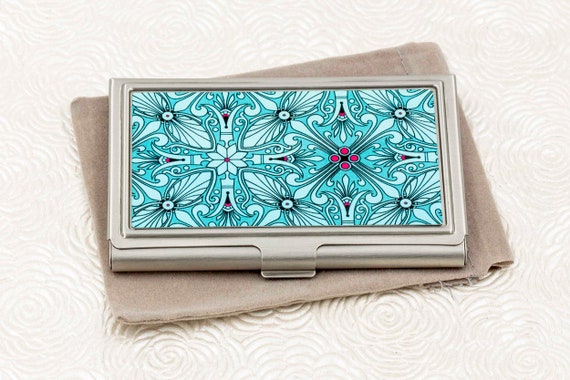The image displays a satin silver tin case, which might be a compact or cigarette case, featuring an intricate turquoise and light blue design reminiscent of dragon wings or Art Deco motifs. The cover also highlights a four-sided flower with four red berries at its center. This case is placed atop a light gray or brown carrying satchel, all set against a textured white background adorned with repetitive floral patterns, akin to quilted material. The case has a distinctive lift and pull-up clip at its center, adding to its elegant and vintage appeal.